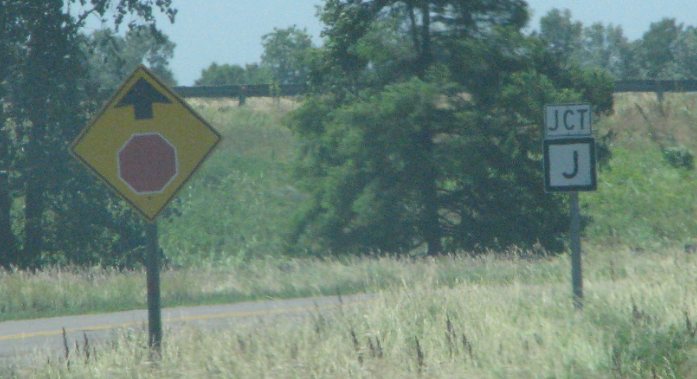A grainy photo, likely taken from a moving vehicle, captures a rural or possibly mountainous area with dim, diffuse lighting. In the foreground, a two-lane highway stretches ahead, flanked by tall grass and dense greenery. On the left side, a yellow diamond-shaped sign warns of a stop sign up ahead, with an arrow pointing up towards the red stop sign. Towards the right, there’s a JCT sign with a large 'J' beneath it, indicating a junction. The scene includes clear skies and a guardrail, with glimpses of flat towers in the distance. The area is dotted with light green shrubs and towering trees, adding to the scene's rural ambiance.